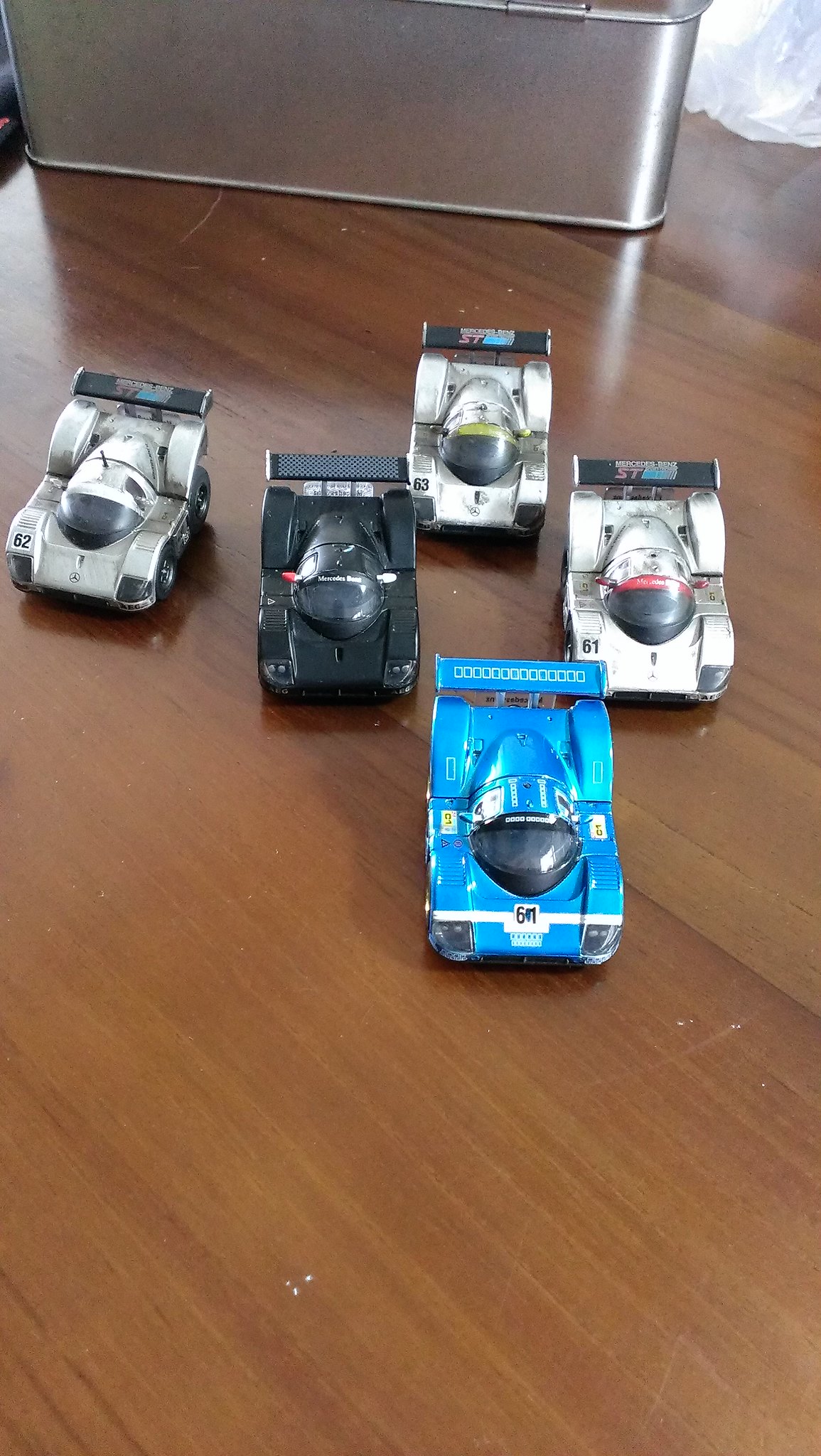This photograph showcases a collection of five miniature Le Mans-style race cars arranged on a brown wood grain surface, possibly a floor or table, that displays signs of slight scuffing. The cars, which resemble Hypercars or futuristic Formula One vehicles, are slightly out of proportion, appearing somewhat chubby with exaggerated features. Each car has a distinct number: 61, 62, and 63. From left to right, the first car is a silver-gray car with black detailing and the number 62. Next, there is an all-black car, centrally positioned. Behind it is another silver-gray car marked with the number 63. Moving right, there's a silver car numbered 61 with black accents. Lastly, at the forefront to the right is a vibrant blue car with a matching blue fin at the back and a black center pod. All these cars share common features such as covered wheels, single cockpits resembling jet canopies, and rear fins. In the background, there appears to be a cabinet or container, adding context to the setting. The overall scene highlights the detailed and distinct characteristics of these toy race cars in a realistic yet slightly whimsical manner reminiscent of Hot Wheels designs.